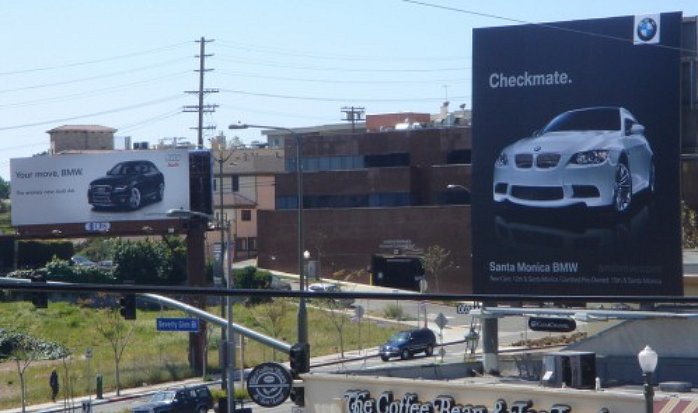The photograph captures a bustling city street on a clear, cloudless day, viewed from a high vantage point, possibly a rooftop. Dominating the scene are two prominent billboards that are partaking in an advertising duel. On the left, a large billboard showcases a black car with the bold, competitive text "Your Move, BMW." This billboard suggests a friendly rivalry, and it's likely an Audi ad challenging BMW.

Across the street on the right side, a prominent vertical billboard displays a white car with the triumphant caption "Checkmate" along with the tagline "Santa Monica BMW," indicating BMW's bold rebuttal. Enhancing the competitive narrative, the BMW billboard features contrasting colors of blue and white, and silver wheels on the car depicted, emphasizing its sleekness.

Below these billboards, the street teems with activity. Trees, a fenced-off grassy area, and a clean sidewalk can be seen to the left. The buildings lining the street include a notable establishment named "The Coffee Bean," catering to urban dwellers. Electrical power lines stretch across the scene, and a brown brick structure and a parking garage are visible in the backdrop. Cars navigate the street, underscoring the everyday hustle of the city. The photograph, rich in urban details and advertising dynamics, captures a moment brimming with both vehicular and commercial energy.